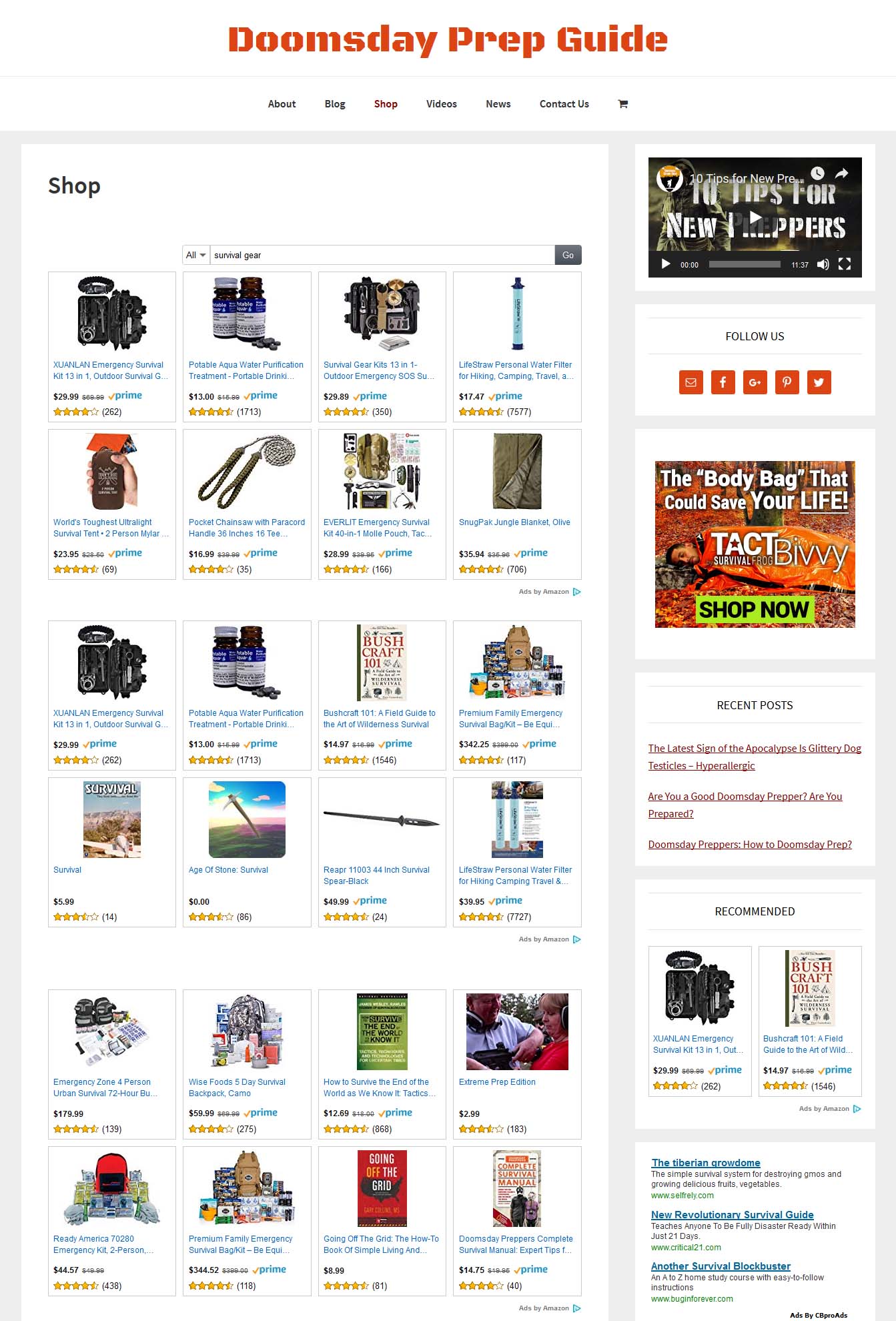The website, titled "Doomsday Prep Guide," features a navigational menu at the top with various tabs: About, Blog, Shop (currently highlighted), Videos, News, and Contact Us, along with a Shopping Cart icon. Below this menu, the main frame displays the "Shop" section, organized in a grid format comprising four columns by six rows. The products showcased are specifically designed for doomsday preparation and include items such as survival kits, medicines, books like "Bushcraft 101: How to Survive in the Wild," survival guides, first aid kits, and a book titled "Going Off the Grid." Additionally, a side panel highlights various ads, recent blog posts, and recommended shop items, enhancing the site's overall utility for those interested in emergency preparedness.